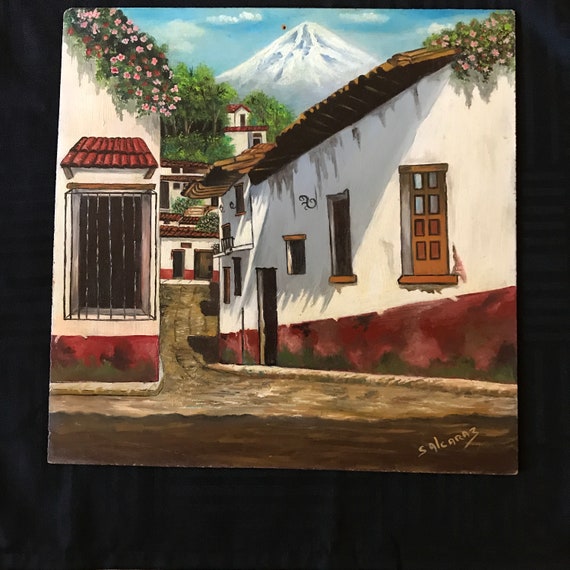This image features a detailed hand-drawn piece of art on a canvas set against a black background. The artwork, created by an artist whose signature reads "SALCARAZ" at the bottom right corner, portrays a charming Mexican-style village. The central scene is a narrow brown pathway flanked by two beige-colored houses with red trim at the bottom. The house on the left has a barred window, while the house on the right, angled slightly, features both windows and a doorway. Pink flowers with green leaves grace the rooftops of these homes. In the distance, similar beige buildings populate the landscape, leading the eye toward a majestic snow-capped mountain peak that dominates the background under a blue sky with white clouds. The vibrant greenery of surrounding trees further enhances the idyllic outdoor scenery depicted in this oil painting style artwork.